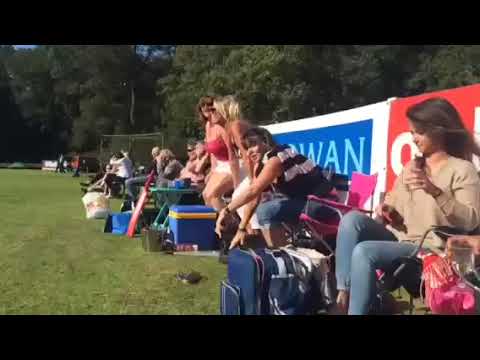In this photo of an outdoor daytime event, possibly a sporting event, a group of people, likely parents, are seated along a fence line in a park. The scene features an array of colorful banners, hinting at sponsorships, attached to the fence. The people are either sitting in foldable chairs, some with drinks in hand and coolers and small tables nearby, or standing around engaging in conversation. Prominently, a woman in a tan shirt and blue jeans sits in front of her tote bag, while another woman further down the line wears a black and white sweater with blue jeans. Several others dressed in shorts suggest a warm-weather setting. Beyond them, more spectators can be seen, although they are too far to discern clearly. The image also shows tree lines in the background, adding to the lush greenery of the park. The predominant colors in the photo include various shades of blue, green, pink, red, yellow, black, white, and grey.